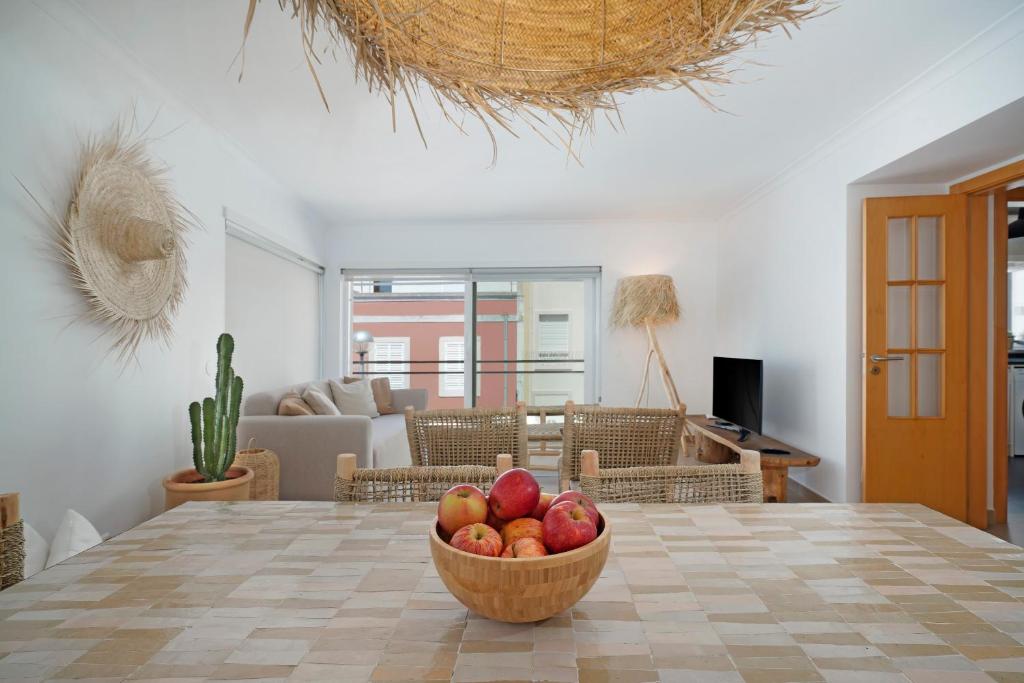This vivid color photograph captures the cozy interior of an apartment living room. In the foreground, a dining table with a distinctive brown and beige checked pattern is adorned with a wooden bowl filled with red apples. Two chairs with organic designs crafted from rope and wood are tucked neatly under the table. Adjacent to the table stands a cactus in a pot, adding a splash of greenery to the scene. Centered against the wall, a gray sofa, embellished with four pillows, faces a wooden TV stand holding a flat-screen television. A sliding glass door behind the sofa reveals a view of buildings across the street, lit by daylight. The bright, white interior walls are complemented by an array of unique decorative items, including a light with a wooden cover, a large circular hat on the left wall made from dry twigs and bushes, hanging like a Mexican sombrero, and an impressive circular twig structure fixed to the ceiling. The room exudes a blend of rustic and modern elements, further enriched by the orange French doors on the right, one of which is partially open, offering a glimpse into the adjoining room.